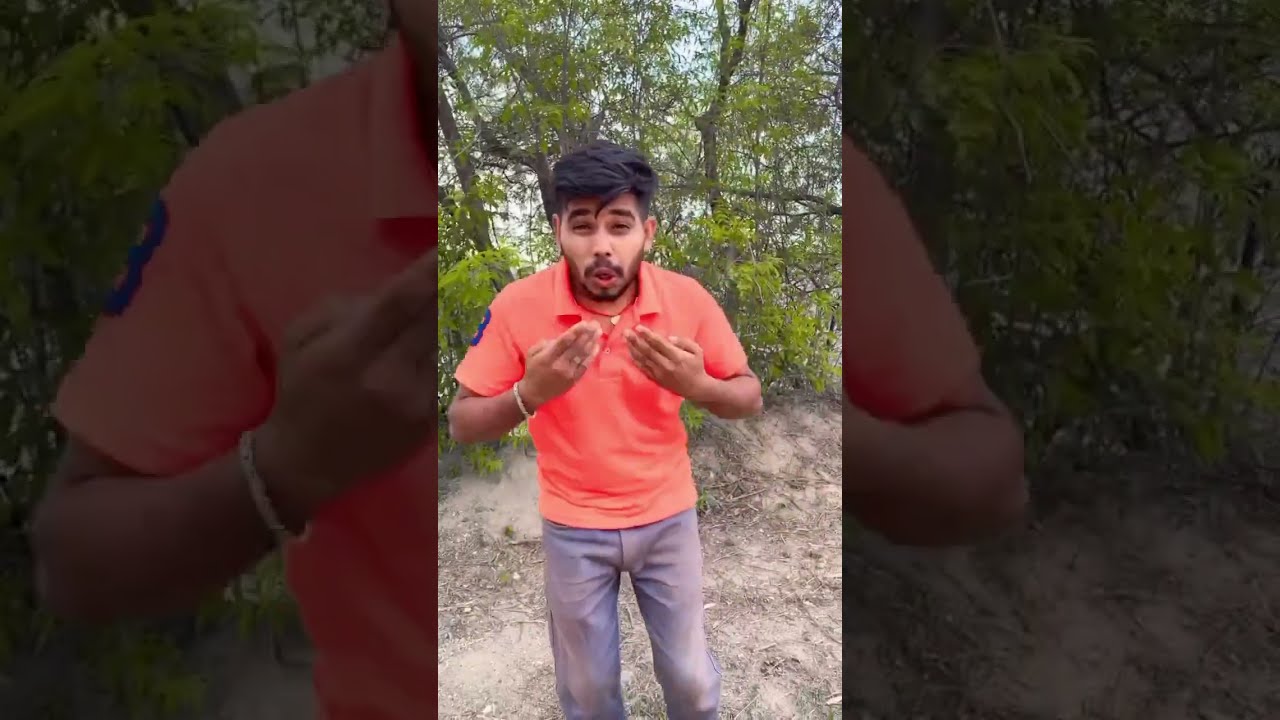This is a detailed photograph of a man standing outdoors, set against a forest backdrop. He has dark, black hair, a mustache, and a beard, with brown skin. The man is dressed in a red-orange t-shirt that seems to have a blue number on one sleeve and is paired with blue jeans, which appear a bit dirty and have a grayish-brown tint. His wrists feature a golden bracelet and a necklace can be seen around his neck. He is leaning slightly forward with both hands raised to chest level, his palms facing him, and makes a peculiar expression with his face, his mouth forming an "O" shape and his eyes squinted as if trying to speak or shout. The ground beneath him is brown soil, and the background shows trees with green leaves, under a clear blue sky. The vertical rectangular image has prominent borders on the left and right sides, which are blown-up and faded versions of the central image, effectively creating a unique frame.